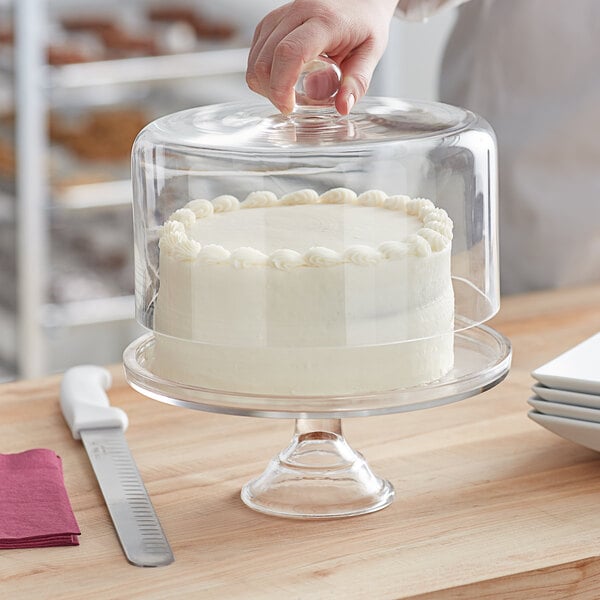In the photograph, a person dressed in white is either placing or removing the dome lid from a pristine, white-iced cake that sits smoothly on a clear glass cake stand. The cake is impeccably smooth on the top and sides, with a decorative seashell border of icing along the edges. The cake stand rests on a natural-tone wooden table, accompanied by a cake knife with a white handle. To the side, there are burgundy (or magenta) napkins and partially visible white square plates. In the blurred background, you can see shelving that appears to hold additional sweet treats, though they are not in clear focus.